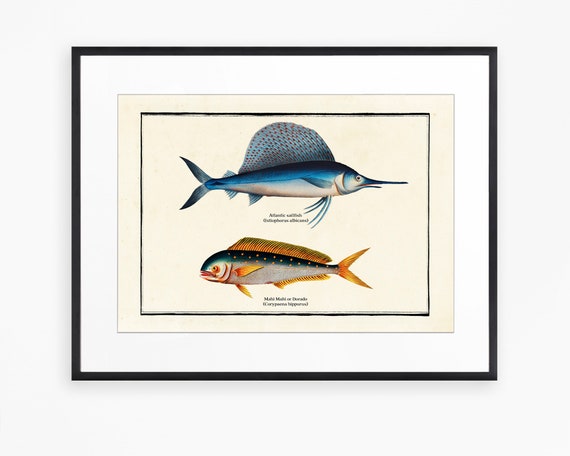This image is of a framed print, resembling an old painted illustration typically found in nature books, depicting two distinct fish on a mostly white background with an off-white border, enclosed by a black-bordered matte. The top fish is identified as an Atlantic sailfish, characterized by its elongated blue body with a large, round dorsal fin that is wider and taller than its body. The sailfish has a sword-like nose, a blue upper body, and a white belly. The bottom fish is a mahi-mahi, featuring a more rounded head and a long body. It displays a striking combination of colors with a blue top speckled with golden spots, a silver underside, and vibrant yellow fins including a long fin extending down its back. Both fish have forked tails and detailed features that suggest biological names in Latin beneath them, though the resolution prevents clear reading.